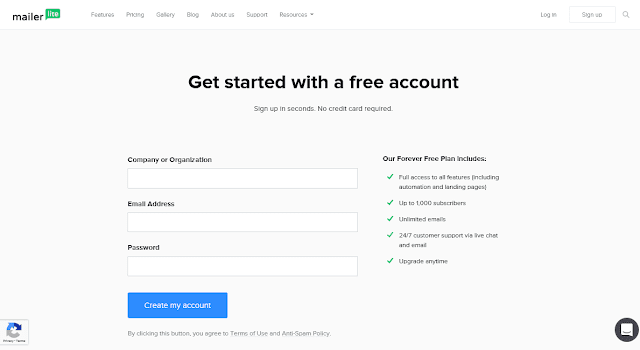The image is a screenshot from the MailerLite website, showcasing the option to set up a free account. At the top of the page is the MailerLite logo, with "Mailer" in bold letters and "Lite" in white letters inside a green box. The navigation bar includes the options for Features, Pricing, Gallery, Blog, About Us, Support, and Resources, with a dropdown menu. On the right side of the navigation bar, there are options for Log In, Sign Up, and a search icon represented by a magnifying glass.

Central to the image, on a gray background, is a call-to-action text that reads "Get Started with a Free Account. Sign Up in Seconds, No Credit Card Required." Below this, a section highlights the benefits of the "Forever Free Plan," mentioning full access to features, including automation and landing pages, support for up to 1,000 subscribers, unlimited emails, and 24/7 customer support via live chat and email. It also notes that users can upgrade at any time.

To the left, a sign-up form is displayed with fields for "Company or Organization," "Email Address," and "Password." Below the form fields is a blue button labeled "Create My Account" in white text. Underneath the button, a disclaimer states, "By clicking this button, you agree to our Terms of Use and Anti-Spam Policy."